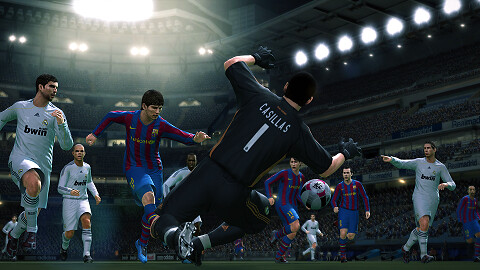This is a detailed screen capture from the FIFA soccer video game, showcasing a highly dynamic moment on the field. The focal point is a player named Casillas, as indicated by the white letters and a large number one on the back of his black uniform. Casillas, who has dark hair and is equipped with black gloves, appears to be diving or falling backwards, with his arms outstretched and the bottom of his right cleat visible. His left foot is bent back behind him, and he is angled towards the right. 

In the background, there are players incoming, who wear blue and red-striped jerseys paired with blue shorts and blue cleats. One of these players, positioned to the left, seems to be kicking a ball towards the goal. The soccer ball, mainly white with blue and red details, is seen in the air towards the right side of the image, just underneath Casillas’s outstretched arm. 

Additional players in white uniforms are also visible; they wear white shorts, long-sleeved shirts, and tall socks, and appear to be running towards Casillas, likely attempting to regain control of the ball. Further in the distance, the crowded stands and the brightly lit top of the stadium punctuate this action-packed scene, emphasizing the grand setting of the game.